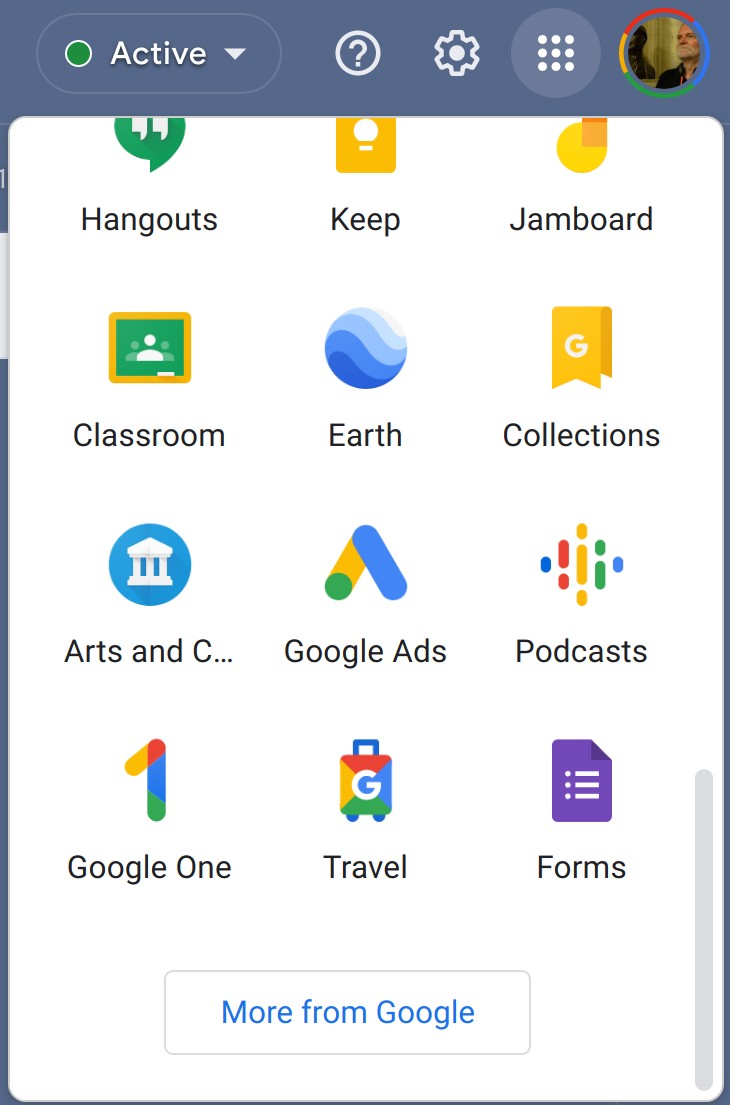Screenshot of a Google Options Panel on a Smartphone

In the image, there's a screenshot displaying a Google options panel on a smartphone. The user interface features a blue header with the label "Active" accompanied by a green dot and a dropdown arrow, all encapsulated within a thin capsule line. To the right of the header are a question mark inside a circle, a gear icon, a grid of nine dots, and a user profile icon. The profile displays a picture of a middle-aged man with a short grey beard, looking off to the left.

Below the header, the tops of various Google app logos are slightly cut off, indicating the panel has been scrolled down. The scrollbar on the right is at the bottom. The interface shows a grid of three columns across and four rows down, featuring different Google services. At the bottom, there's a button labeled "More from Google."

Here are the visible Google services and their associated icons:
1. **Hangouts** - A green speech bubble with quotation marks inside.
2. **Keep** - A Yellow box with a light bulb inside.
3. **Jamboard** - An abstract yellow and orange icon.
4. **Classroom** - An icon resembling a chalkboard.
5. **Earth** - A blue and white swirling globe.
6. **Google Collections** - A 'G' with a badge and a bookmark icon.
7. **Google Arts & Culture** - An icon of a pillared building.
8. **Google Ads** - A chevron-like logo.
9. **Google Podcasts** - Multicolored dashed lines representing sound waves.
10. **Google One** - The numeral "1" with a multicolored stripe.
11. **Google Travel** - A suitcase icon.
12. **Google Forms** - An icon representing a document with checkmarks and lines.

This panel provides quick access to a variety of Google applications and services directly from the smartphone interface.